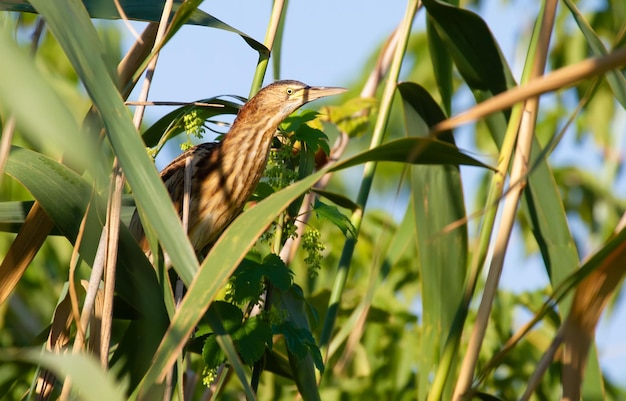This horizontally rectangular, full-color nature photograph captures a close-up of a bird nestled in dense underbrush on a sunny day. The background features a blue sky peeking through the array of plant life, composed of long green leaves and brown stems topped with green foliage. Positioned on the left side of the frame, the bird is in profile, looking right. It has an elongated neck and is adorned with alternating lighter and darker brown stripes along its body and underbelly. The bird's throat is lighter in color, and it sports a dark stripe on the top of its head. Its beak, which is yellowish with a black base, extends prominently from its head. Only one of its small eyes is visible, adding to the detailed texture of its striped feathers. The tail feathers, which also bear brown and white stripes, peek out slightly.